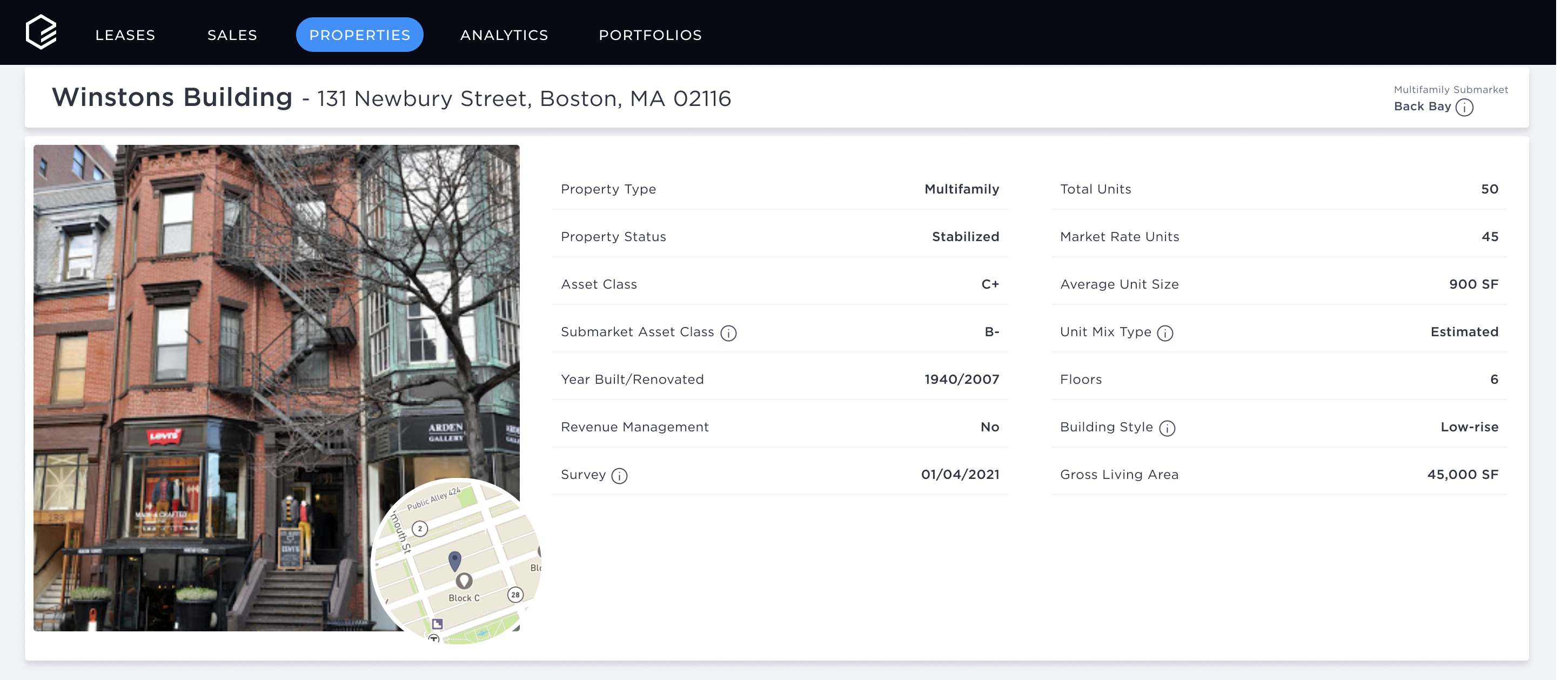Screenshot of a property management website showcasing a detailed view of the Winston Building located at 131 Newberry Street, Boston, MA 02116. At the top, a black navigation banner displays menu options for Leases, Sales, Properties, Analytics, and Portfolios, with the Properties option highlighted in a light blue oval, indicating the current section. Beneath this, a photograph of the Winston Building is displayed alongside a small circular map excerpt showing its location.

On the right, occupying 65% of the screen, there's a comprehensive information panel on the property. This section lists 14 key details including Property Type, Property Status, Asset Class, Total Units, Market Rate Units, Floors, Building Style, and more, all presented against a clean white background with basic black text. The website serves as a resource for accessing detailed information about various real estate properties.